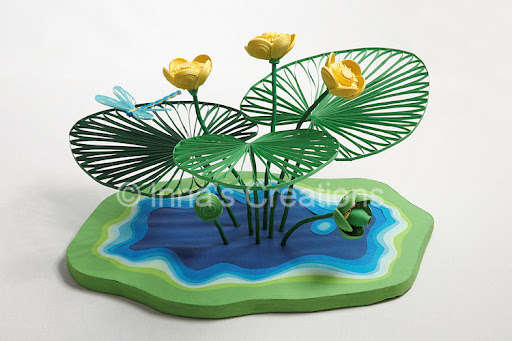This is a detailed art sculpture set against a light blue background. The sculpture features a green, oblong base with a wavy outer edge, resembling a miniature pond. The center of the base is designed to look like a body of water, featuring concentric rings ranging from white and light blue to dark blue, giving a shiny, possibly varnished appearance. Emerging from this pond are delicate structures mimicking lily pads, crafted from green wire, creating see-through, round leaf shapes on slender stems. Among these leaves, there are three ranging in color from light to dark green. On the dark green lily pad on the left side, a tiny blue dragonfly is perched. Adding to the lifelike pond scene, there are three vibrant yellow lilies positioned at the top of the sculpture in various directions, along with two smaller lily buds on stems near the base, extending out of the water-like center. This intricate artwork evokes the serene and natural beauty of a lily pond.